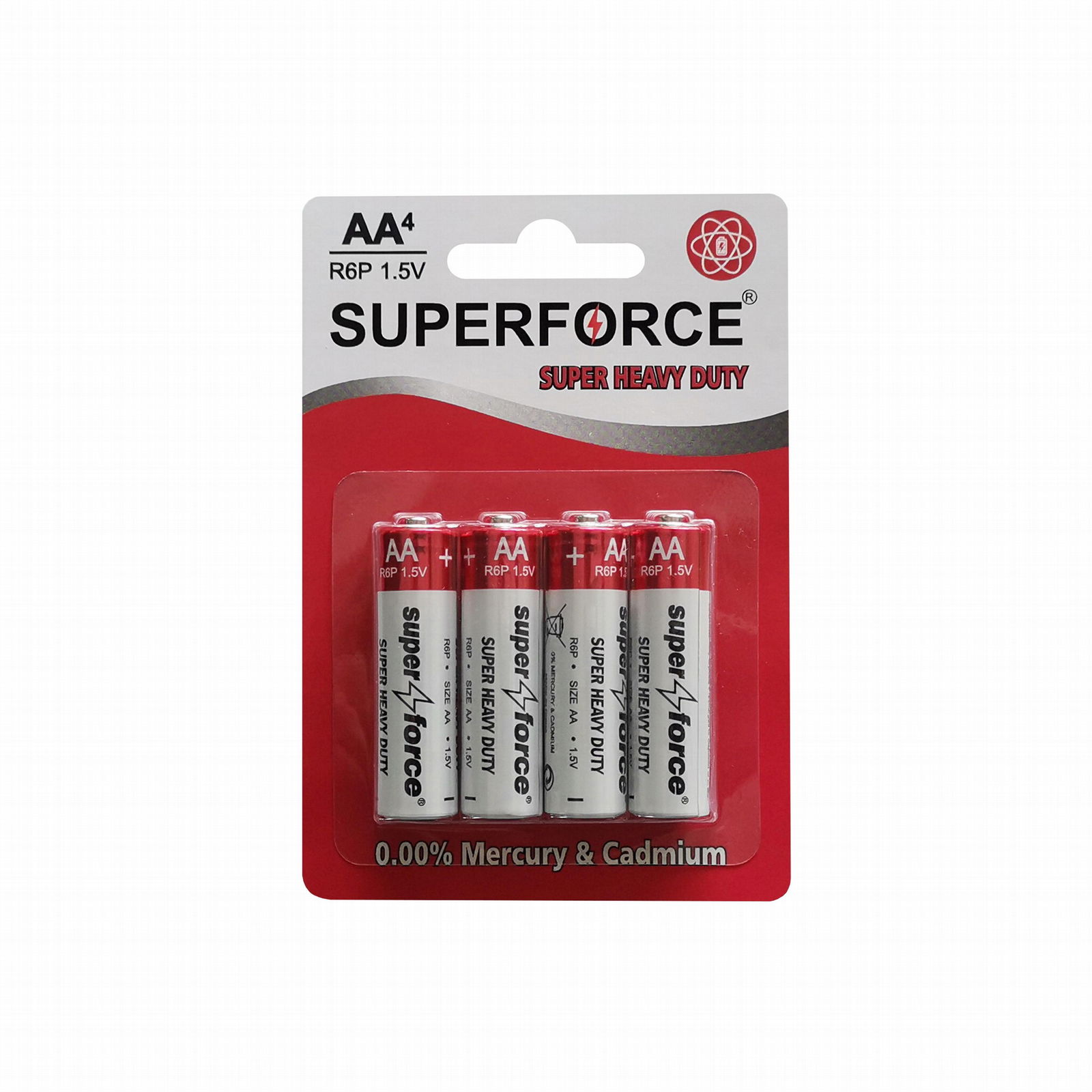Detailed Caption: 

This image showcases a package of four AA batteries, measuring approximately six inches in height. In the upper left corner of the packaging, "AA" is prominently displayed in capital letters, denoting the battery type. Positioned diagonally to the right corner of these letters is the number "4," which is underlined. Beneath this, the alphanumeric code "R6P 1.5 V" is inscribed, indicating the battery specification and voltage. 

To the right of these details, there is an open area of the battery case which features a distinctive design. This includes a series of overlapping ovals rendered in white, within which resides a small red circle. Below this intricate design, the brand name "SUPER FORCE" is written in all capital letters. The "O" in "FORCE" is accentuated by a red lightning bolt. Additionally, the terms "SUPER HEAVY DUTY" are prominently printed in red beneath the brand name.

The four AA batteries are partially visible within the packaging. The tops of these batteries are colored red and are labeled with "AA" alongside a positive symbol. The bottoms are white and bear the brand name "SUPER FORCE," with the iconic lightning bolt symbol placed between the words "SUPER" and "FORCE." At the bottom of the packaging, it states "0.00% mercury and cadmium," confirming that the batteries are free from these hazardous materials.